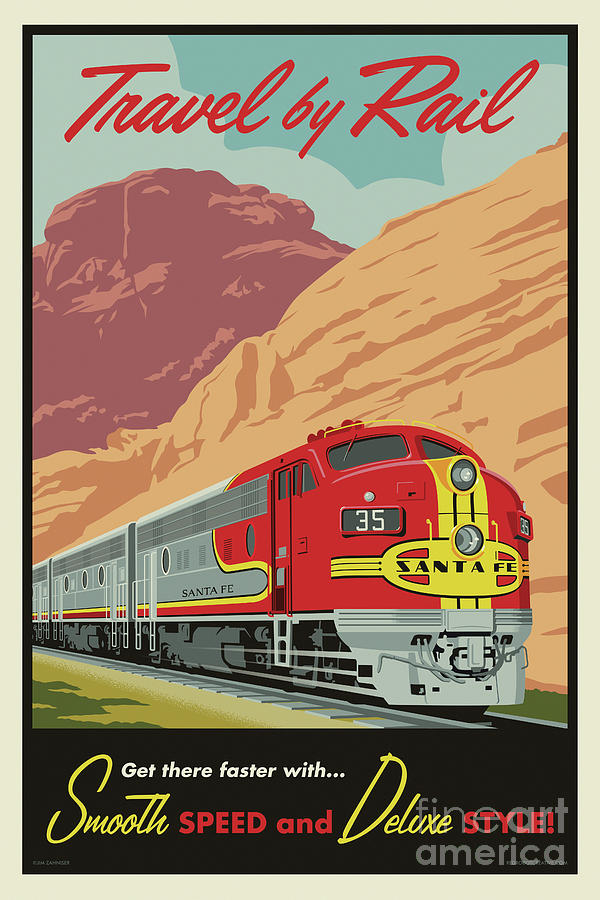This promotional poster, reminiscent of a 1950s advertisement, showcases a sleek, Santa Fe branded train speeding through a picturesque canyon. At the top, in bold red cursive lettering, it proudly declares, "Travel by Rail." The train itself is a striking blend of colors: its front showcases a vivid red with a yellow stripe and the iconic yellow Santa Fe logo emblazoned across it. The engine, marked with the number 35, transitions into soft gray with a continuing stripe of red and yellow along its length, adding to its sleek and modern appeal. The railway winds from the bottom left towards the middle right of the image, against a backdrop of brown and red sandstone formations. The scene is enclosed in a dual border—beige on the outside and black on the inside. At the bottom, within the black border, a slogan reads, "Get there faster with smooth speed and deluxe style." The words "smooth" and "deluxe" shine in gold, while "speed" and "style" boldly stand out in red. Additionally, a subtle watermark in the bottom right-hand corner reads "Fine Art America," with "Fine" in thin print and "Art America" in bold. The overall effect is a colorful yet sophisticated depiction that captures the essence of luxurious and efficient rail travel.